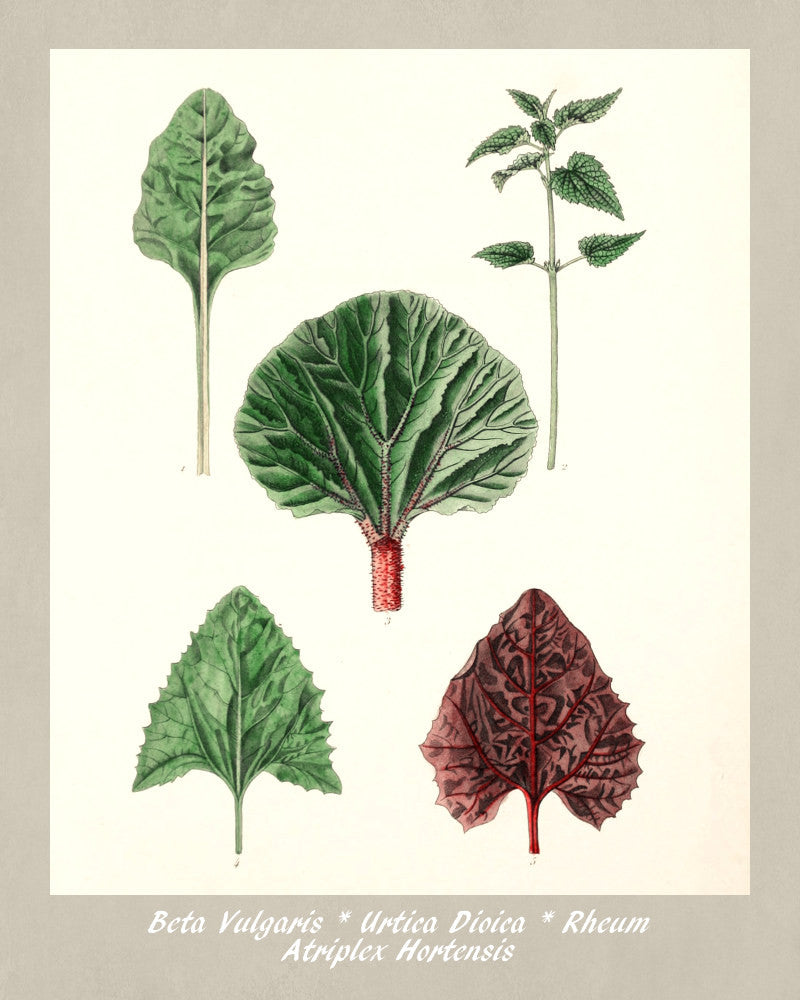The image is a detailed poster featuring illustrations of five different plant leaves, arranged in a cross pattern. The background of the poster is cream-colored, framed by a light gray border. At the bottom of the poster, botanical names are inscribed in white text: Beta vulgaris, Urtica dioica, Rheum, and Atriplex hortensis. Each leaf is meticulously illustrated, likely using colored pencil.

The positions of the leaves are as follows: on the bottom left is a green, triangular-shaped leaf with a tall stem; directly to the right is a wide, purple leaf with red undertones. The center leaf is large and fan-shaped, green with a reddish stem. The top right leaf is characterized by a long stem sprouting multiple textured green leaves, while the top left leaf showcases a singular, elongated green leaf with a rounded triangular shape. Each leaf is marked with a number for identification.